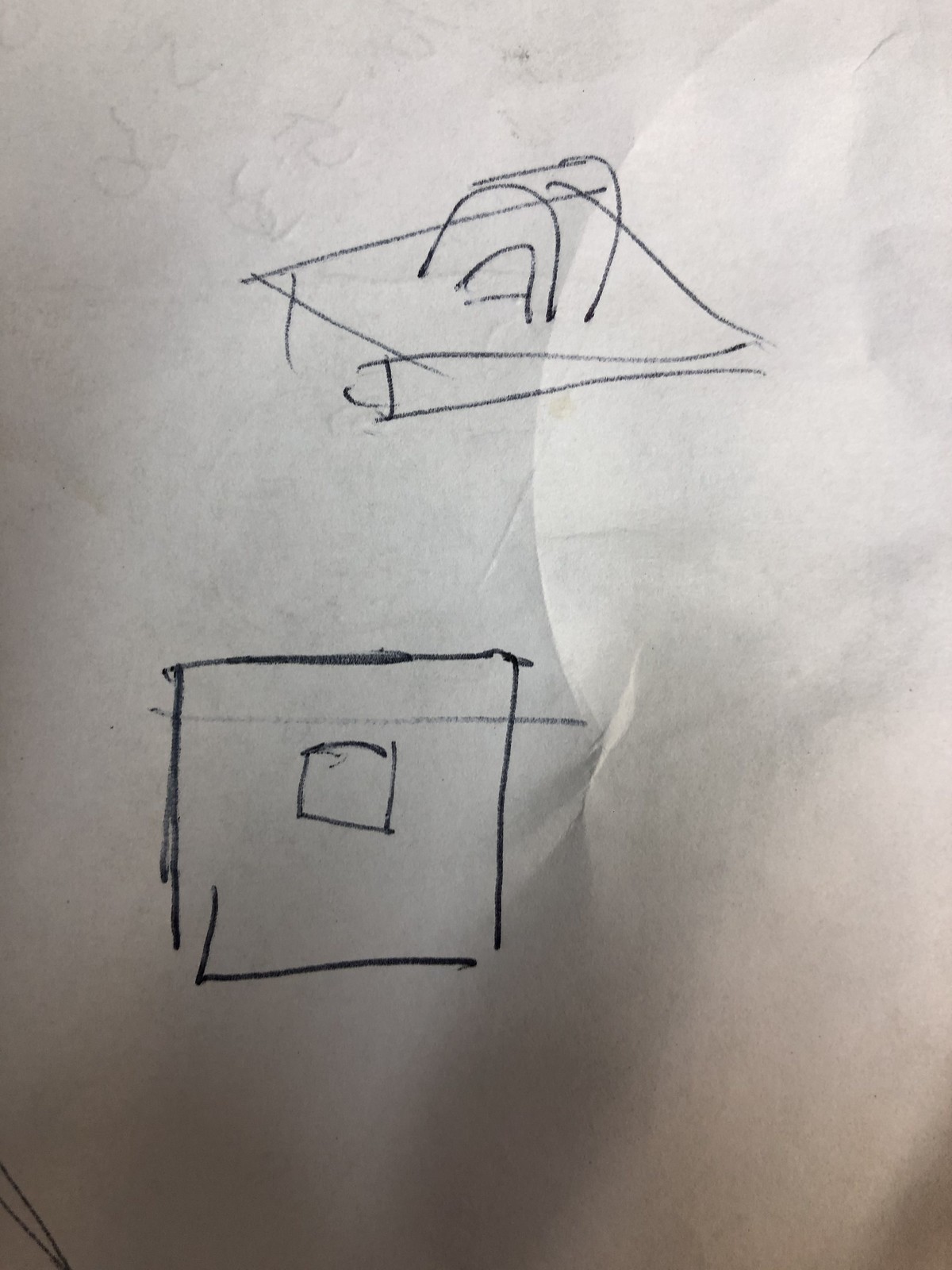This is a photograph capturing a hand-drawn illustration on a sheet of white paper. The drawing, executed hastily using either ink or a magic marker, consists of two distinct but possibly related sections.

The upper part of the drawing features a square with an arch on top and another arch beneath it, resembling the profile view of a structure such as a roof or possibly a chimney. The line work appears quick and unrefined, suggesting it was sketched spontaneously.

Beneath this, there is a second drawing: a large square that contains a smaller square within it, topped by a horizontal line. This depiction might suggest a top-down view of the same structure illustrated above, with the central square potentially representing the upper arch from the first drawing.

Overall, the composition seems to be a study of a simple structure from different perspectives—one side profile and one aerial.